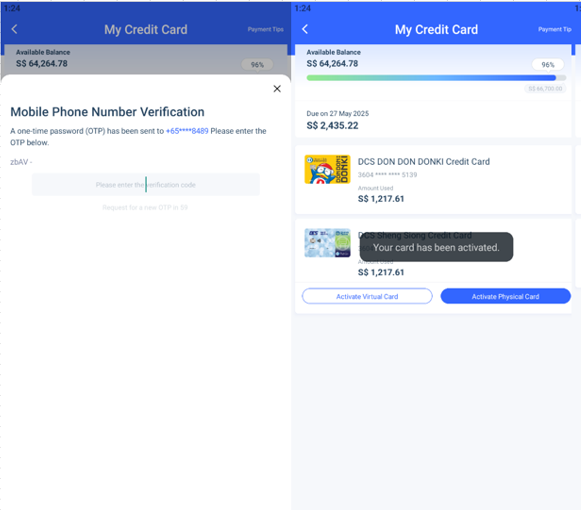The image shows two side-by-side screenshots from the "My Credit Card" section of a mobile app. The top of each screenshot displays standard phone information including the time, with a blue banner labeled "My Credit Card."

On the left screenshot, the user's available balance is displayed. A pop-up box prompts mobile phone verification, indicating a one-time password (OTP) has been sent to a specified telephone number (highlighted in blue). The user is instructed to enter the OTP in a designated grey box below the code.

The right screenshot features the full "My Credit Card" page. At the top, the available balance is once again displayed. Below it, a bar graph marked in green and blue indicates 98%. The due amount of $2,435.22 is listed, with a payment deadline of May 27th, 2025. Further down, two credit cards are shown with their corresponding usage amounts. Over the second credit card, a black pop-up states, "Your card has been activated." Below this, options to activate either a virtual card (on the left) or a physical card (on the right) are presented.